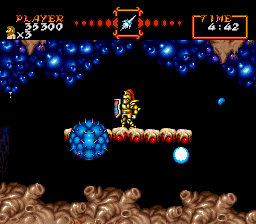This image captures a video game screen immersed in an intense gameplay moment. The background predominantly features a dark, black canvas, setting a dramatic tone. In the top-left corner, the word "Player" is displayed in vibrant orange and yellow letters. Just below it, the player's score, "35300," is shown, followed by an indication of remaining lives, noted as "×3," accompanied by a small avatar icon.

On the top-right side, the word "Time" is conspicuously presented in bold red and orange letters. Directly beneath this are the numerals "442," which are encased in a striking orange and red rectangular border.

Centre stage, a formidable knight clad in traditional knight's armor takes his stance, gripping a shield. He stands poised on a platform that's a blend of brown and red hues. To the knight's left, a large, menacing blue ball adorned with red spikes hovers, adding an element of peril and challenge to the scene.